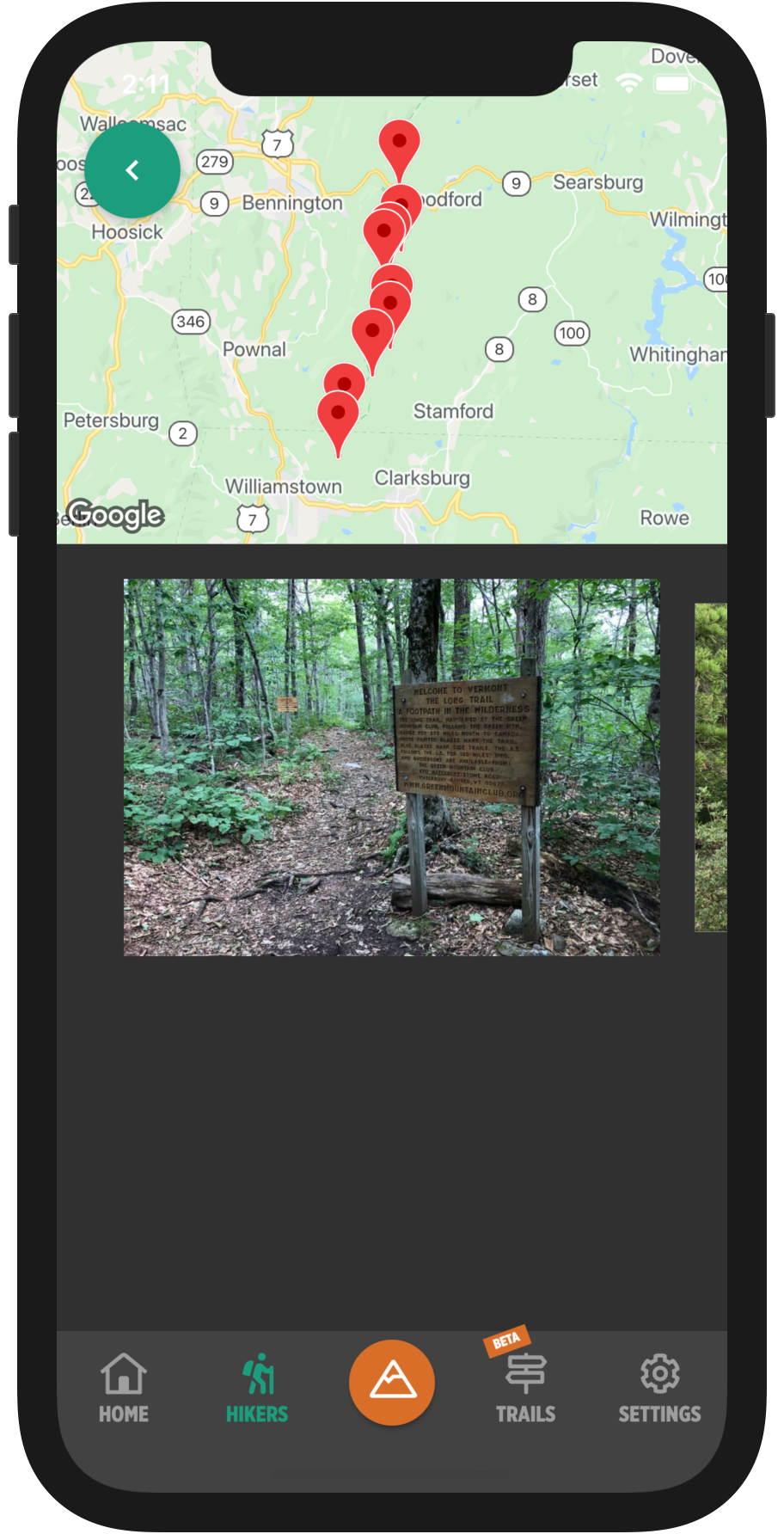This image depicts the screen of an Android phone with a hacker-themed app open. The phone's bottom navigation menu is visible, confirming the Android system. The top portion of the screen displays a GPS map, showing several large brown areas with over ten red pin marks, indicating alert locations. Below the map is what appears to be a photo related to the hitchhiking guide or a specific pin-marked location. The bottom section of the app includes a navigation menu featuring options such as "Home," "Hikers," "Trails" (labeled with an orange "Beta" tag), and "Settings" for app customization. The central orange button likely returns the user to the home menu. The app seems designed for hikers, offering detailed trail information and locations of interest.